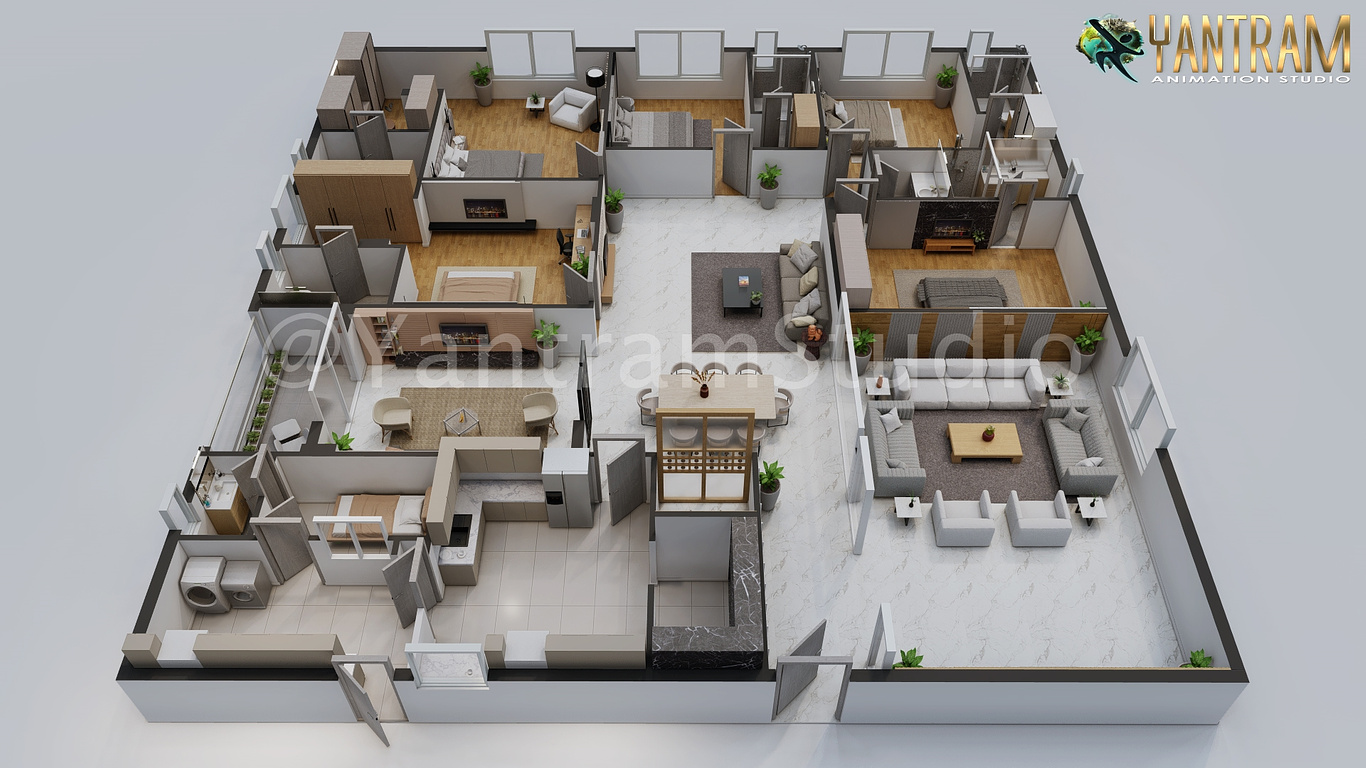This image showcases a highly detailed, angled 3D rendering of a spacious, fully furnished single-story house. The layout includes approximately ten distinct rooms, featuring various types of flooring such as brown wood and white tiles. Notable areas within the house include multiple bedrooms, a living room, a dining area, and an additional sitting area behind the dining space. There is also a well-equipped kitchen and a laundry room. 

Two doors are positioned on opposite ends of the model's front wall; the left door, leading to the laundry room and kitchen, swings inward, while the right door, leading to a living area, swings outward. The back wall of the house is lined with several windows, enhancing the natural light within the rooms. The house is adorned with various pieces of furniture, like sofas, beds, tables, and sinks, making it appear lived-in and practical.

The image background is grey, providing a neutral contrast to the vibrancy and details of the house model. At the top right corner, the logo of Yantram Animation Studios is prominently displayed, with "Yantram" in gold and "Animation Studio" in white. Additionally, there's a small figure of a running person within the logo. Overall, the rendering by Yantram Animation Studios offers a comprehensive and visually appealing floor plan, more advanced than a typical 2D blueprint, and showcases the extensive and intricate design of this large house.